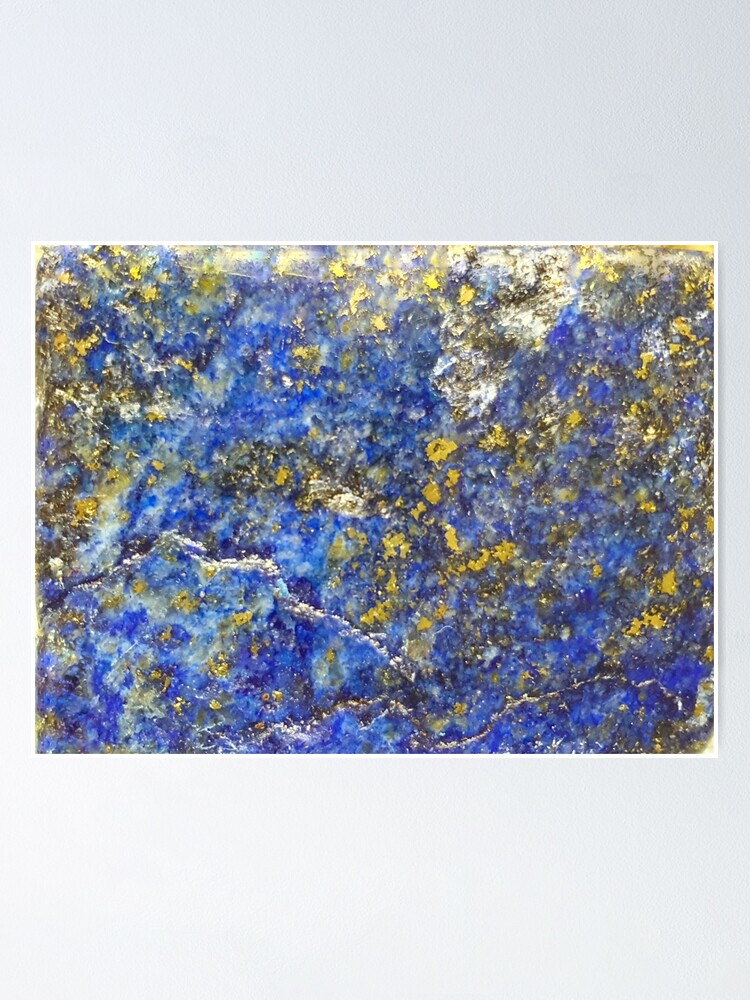This is a detailed description of a striking image that combines various artistic elements. The image predominantly features a blue background interspersed with shades of purple, yellow, and white. The blue could represent a sky or oceanic scene, while the yellow appears somewhat golden, adding a lot of contrast and vibrancy. There are also floral-like dots and foliage-like marks, suggesting branches on a tree with flowers or foliage contrasting with the blue, evoking either nature above ground or aquatic plants.

Central to the artwork are cracks traversing the surface, which is reminiscent of painted cement or stone. One prominent crack starts approximately a quarter up from the left, ascends slightly before curving downwards toward the middle, and splits east and west near the bottom. The west crack extends off the image frame while the east crack rises a bit but doesn't reach the far right.

Additionally, the painting is outlined with a thin white frame and is set against a gray background that casts a shadow, giving it a three-dimensional feel. The texture is noticeable with distinct paint strokes and specks, lending the piece a natural, possibly oceanic impression. Overall, it’s a beautifully intricate composition that combines elements of a floral painting with the textured effect of painted stone, reflecting considerable artistry.